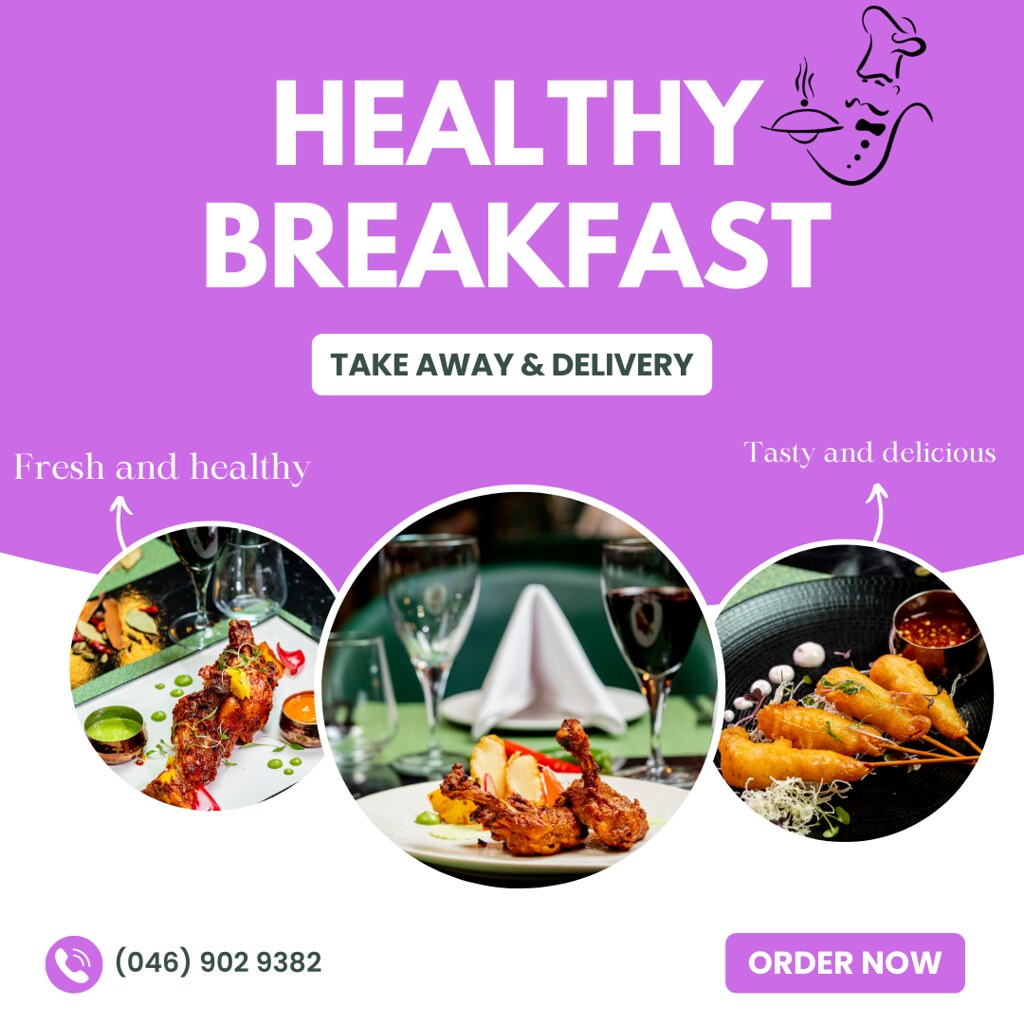The image is an advertisement for a service called "Healthy Breakfast," featuring a prominent purple background. At the top center, bold white letters announce "Healthy Breakfast," with a graphic of a chef's face wearing a chef's hat in the upper right corner. The text beneath this title reads "Takeout and Delivery" in white within a dark background square. Below this, the phrases "Fresh and Healthy" and "Tasty and Delicious" appear in white text on the right-hand side.

The main visual focus consists of three circular photos of various fried food items. The left photo features fried meat on a plate with green and orange sauces, accompanied by an empty wine glass. The center photo appears to display fried shrimp on a plate, with a napkin and a glass of wine in the background. The right photo shows chicken fingers on skewers with a container of red sauce.

In the lower left-hand corner, there is a circular graphic of a telephone followed by the contact number: 046-902-39382. On the bottom right-hand side, a purple rectangle with white text instructs viewers to "Order Now." The advertisement integrates colors like purple, white, black, silver, brown, yellow, orange, and tan to create a vibrant and inviting display.